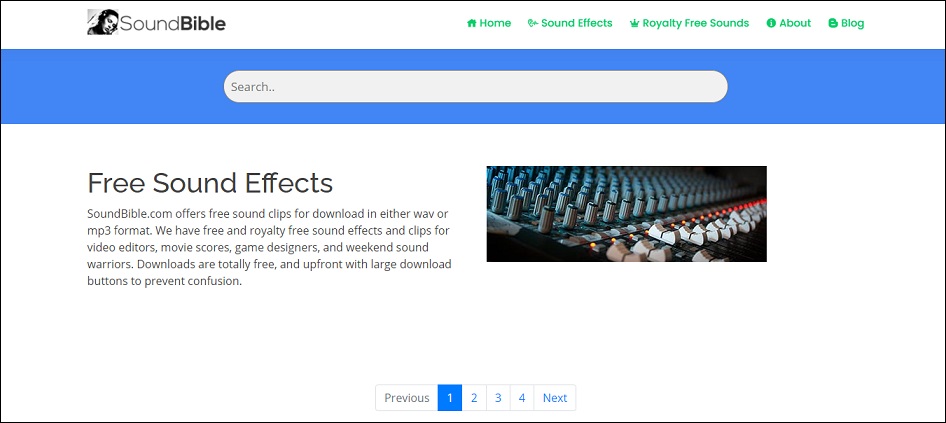This image depicts the homepage of the SoundBible website. 

At the top of the image, there is a white banner featuring the "SoundBible" logo in black letters. Next to the logo on the left, there is a small picture of a man. To the right of the logo, there is a horizontal navigation menu with green letters, displaying the following options from left to right: "Home," "Sound Effects," "Royalty Free Sounds," "About," and "Blog."

Below this navigation menu is a section with a blue background containing a search bar with the word "Search" in grey letters.

Further down, there is a white background with a detailed description of the site's offerings. The text reads: "Free Sound Effects. SoundBible.com offers free sound clips for download in either WAV or MP3 format. We have free and royalty-free sound effects and clips for video editors, movie scorers, game designers, and weekend sound warriors. Downloads are totally free and upfront with large download buttons to prevent confusion."

To the right of this text, there is an image of a keyboard-like device with multiple white buttons. Above the buttons, there are a series of small blue knob-like structures, all set on a black background.

At the bottom-center of the image, navigation options for different pages are displayed, with the word "Previous" on the left and "Next" on the right. Between these, there are numbered boxes for pages 1, 2, 3, and 4, with the box for page 1 highlighted in blue.